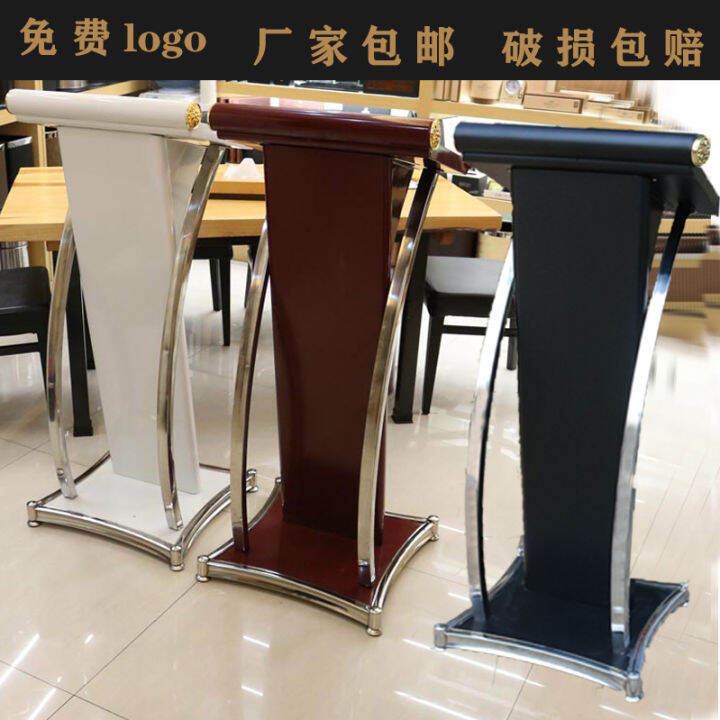The image depicts a product manufacturer's display featuring three modern and minimalistic podiums, which resemble scrolls unfurling from the top to the bottom. These podiums are aligned next to each other, standing on pristine white marble flooring that reflects light from above. The first podium on the left is white, the one in the middle is maroon or reddish-brown, and the podium on the right is navy blue. Each podium features elegant silver trimmings at the base, which artistically lift the "scrolls" up. The silver trims also accentuate the top edges of each stand, drawing attention with their metallic sheen. Above the podiums, there is Chinese text, alongside the word "logo," indicating the commercial or instructional setting. In the background, black chairs and desks reminiscent of a classroom can be seen, adding context to the structured environment.